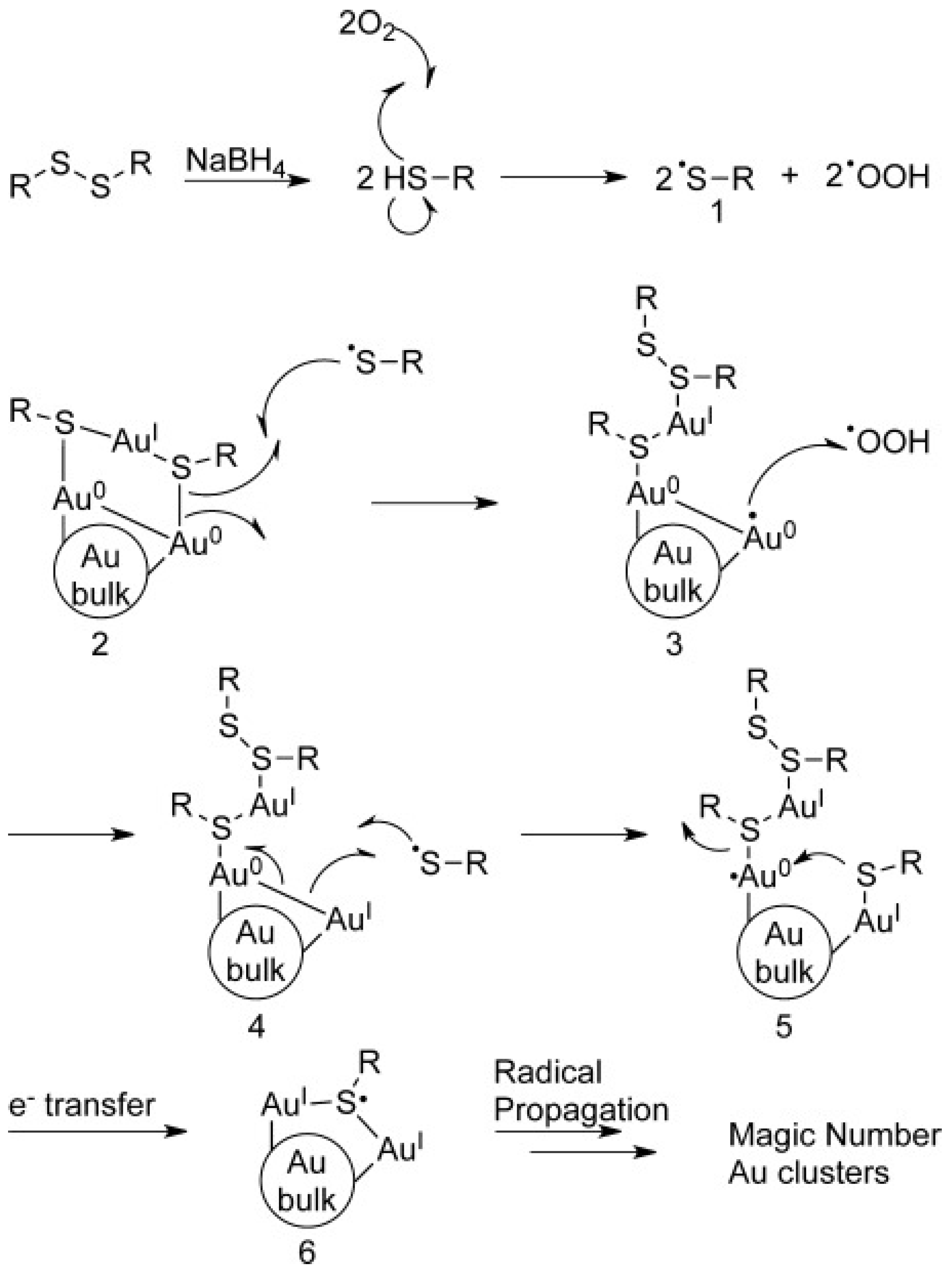The image is a detailed scientific or chemical diagram with a white background and black text, featuring complex chemical equations and descriptions across four horizontally-arranged rows. Each row appears to represent a series of reactions or processes indicated by right-pointing arrows. The first row begins with "RSSR NABH4" and progresses through "2HSR" and "2S-R," ending with "200H." The second row includes more intricate sequences such as "RSSR AU1 RSAU0 AUBulk 2AUO SR RSAU1SRSRAUOAUBULK3AUO 00H." The third row continues similarly with "RSAU1SRSRAUOAUBULKAU1SR4 RSAU1SRSRAUOSRAU1AUBULK5." Finally, the fourth row, labeled “E-Transfer,” transitions through stages like "AU1SRAUBULK6" and concludes with "Radical Propagation, Magical Magic Number AU Clusters." The diagram collaborates various chemical symbols, reaction pathways, and terminologies, culminating in complex AU (gold) clusters.